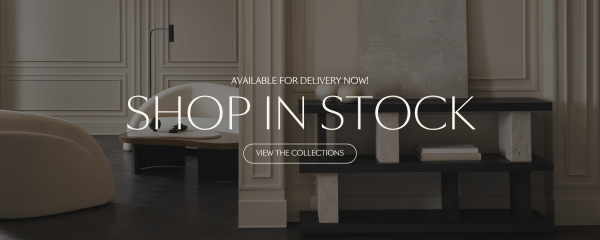The webpage image showcases a user-friendly interface that prominently displays a call-to-action, "Available for Delivery Now," along with options to "Shop in Stock" and "View the Collections," the latter within a clickable white box. The text is rendered in white, set against a background featuring a well-designed interior living space. The scene includes a brown hardwood floor, sleek white chairs, and a stylish wooden table with a black top. The tabletop is adorned with a variety of brick-shaped, white decorative items. Additionally, the setting includes white doors and baseboards, enhancing the sense of a modern, elegant home interior. This layout is indicative of the kinds of high-quality furniture and decor items available for purchase on the website.